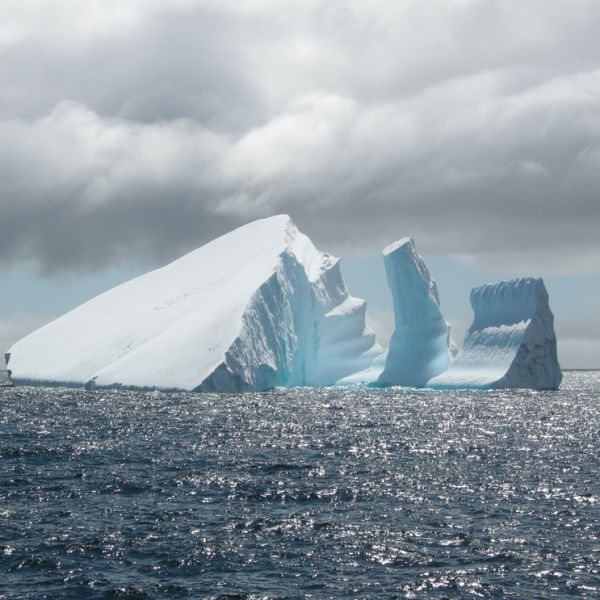This photograph captures a serene scene of three fragmented icebergs floating in the deep blue waters, possibly in the Arctic Sea or near the North Pole. The image is taken from the perspective of a boat, offering a wide view that spans almost the full width of the photo. The largest iceberg on the left has a very flat top and slopes downward, leaning slightly to the left. In the center stands a finger-like piece of ice jutting out, while on the right is a smaller, triangular chunk. Each iceberg boasts a pristine white surface interspersed with hints of light blue in shadowy areas. The calm ocean below them is dotted with tiny highlights reflecting sunlight, indicating a sunlit day despite the dark, barrel-like clouds filling the sky above, suggesting the imminent possibility of a storm.